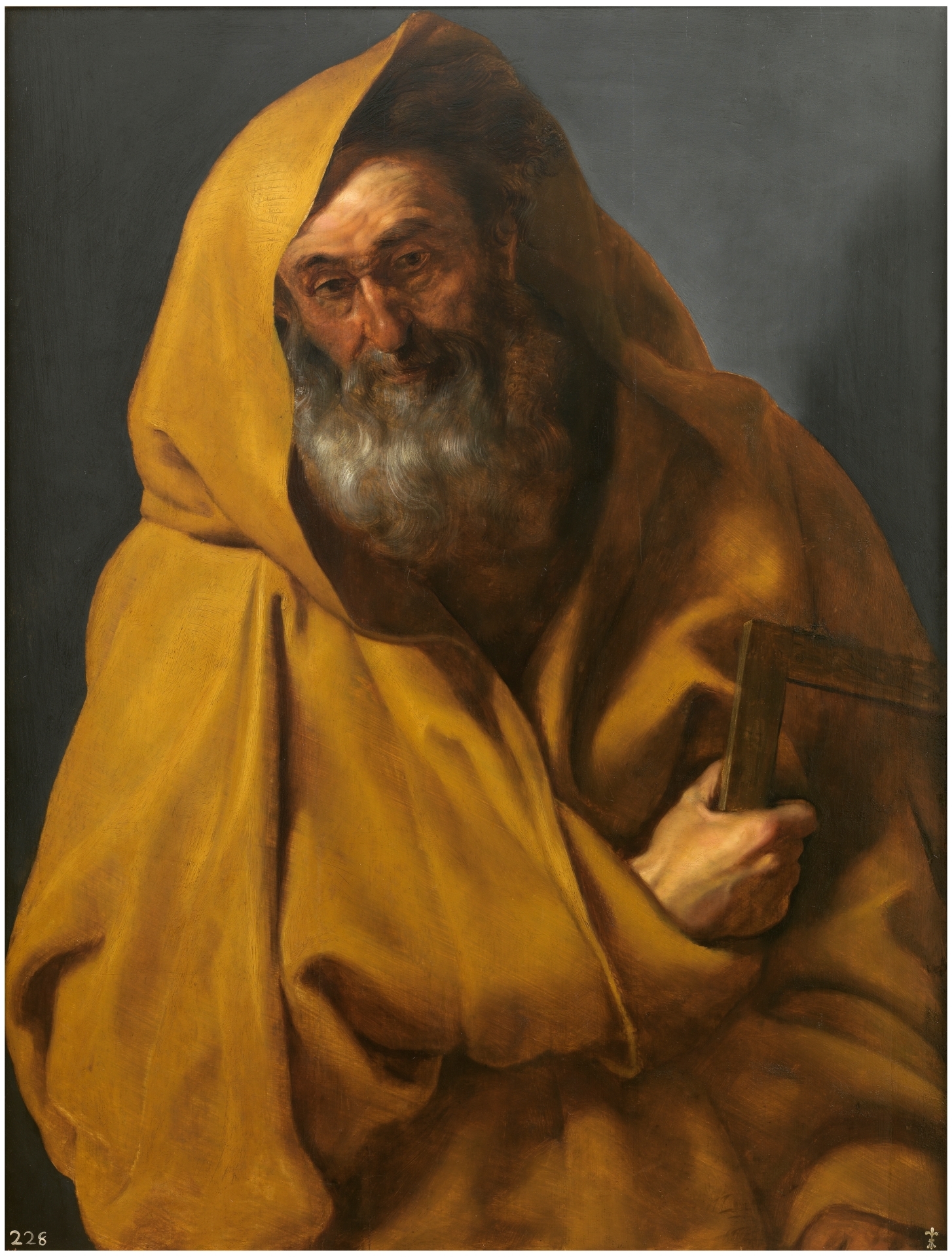This oil painting, numbered 228 and signed by the artist, features an older Caucasian man clad in a large, hooded yellow-brown robe, set against a black gradient backdrop. The man, depicted from the waist up, has a bushy gray beard, a mustache, and short, wild gray hair peeking from under the hood. His weathered face bears lines on the forehead and bags under the eyes. Gazing down towards the lower left, he clutches a piece of wood, angled like the top of a painting frame, in his left hand. His shadow subtly blends into the dark background, adding a haunting, almost ethereal quality to the scene.